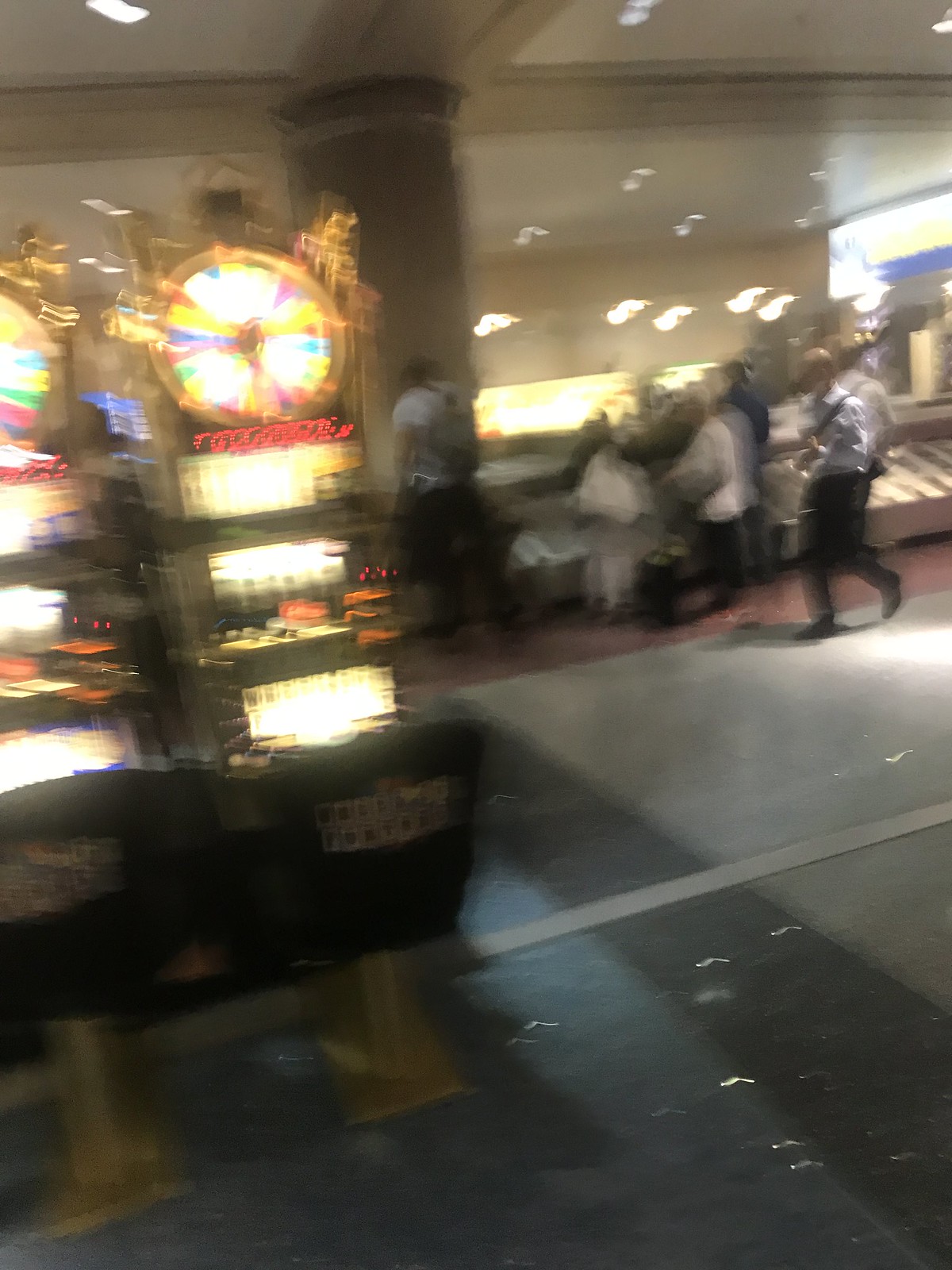In a blurry photograph of an arcade, the focal point is a pair of identical arcade games situated prominently on the left-hand side. The games feature a distinctive design, including a gold circle at the top, adorned with gold trim. The gold circle's perimeter resembles a clock face, with colorful triangles—purple, yellow, blue, and pink—instead of numbers. Below this decorative element, there are red letters that are unreadable due to the image quality. The front of the arcade machines displays horizontal rectangles of white light, interspersed with black lines. The lower section of each machine seems to feature a seating area, possibly a chair, with more unreadable text on it. The arcade's floor is gray with a few stripes, and in the background, some people are walking past indistinct objects. The overall scene is lively but indistinct due to the photograph's blurriness.